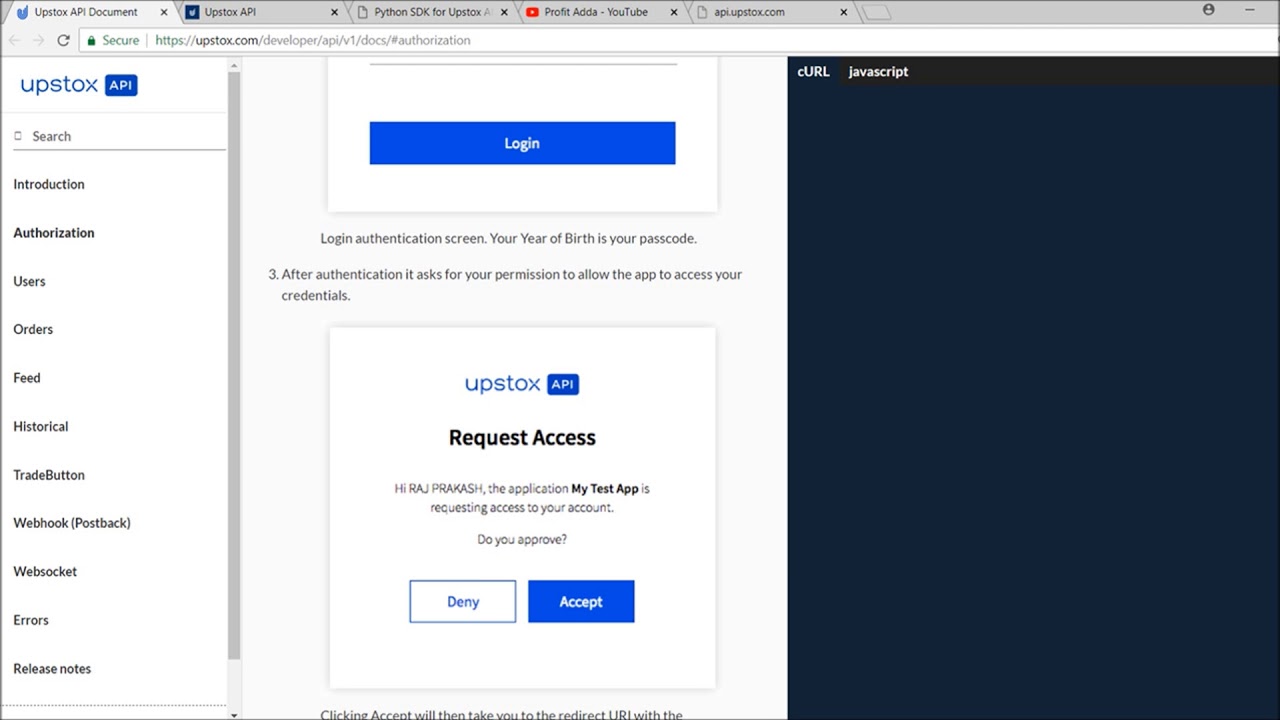A screenshot of a web browser window with multiple tabs open, highlighting various resources related to the Upstox API. The open tabs include "Upstox API Documentation," "Upstox API," "Python SDK for Upstox," and a YouTube video titled "ProfitAdder." Another tab displays an error page with the URL "https://apx.upstax.com." The active tab shows the URL "https://upstax.com/developer/api/vt/docs#authorization," revealing a login authentication screen. At the top of the page, a blue rectangular login button is prominently featured. Below it is a text box explaining that the year of birth is used as a passcode for authentication. The page goes on to ask for user permission to allow the app to access credentials. Further down, a message addressed to Raj Prakash states that "My Test App" is requesting access to his Upstox account, seeking approval.